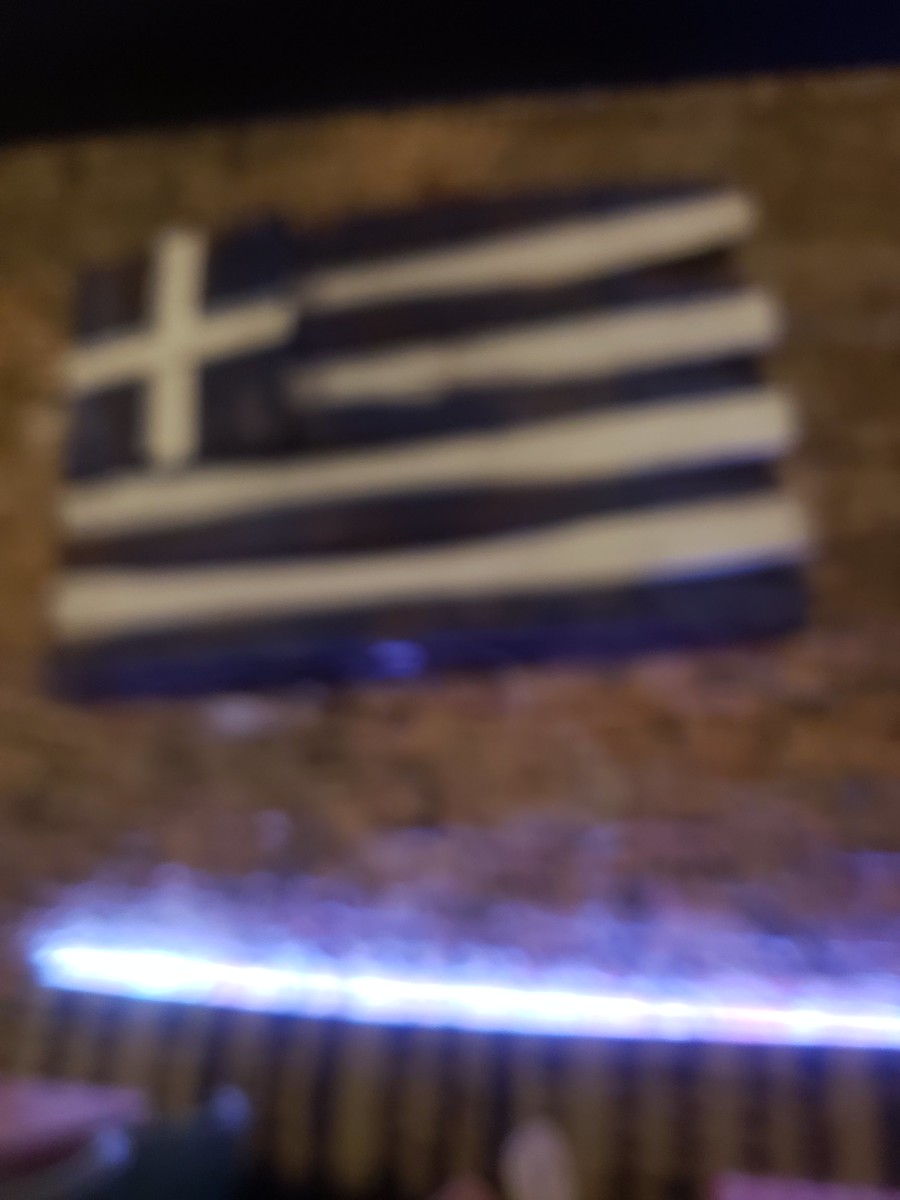The image is an extremely blurry photo, possibly taken indoors, maybe in a bar or restaurant. The main subject is a flag with a unique design: it features blue and white horizontal stripes and a white cross in a blue square located in the top left corner. This resembles an American flag but with a blue field and a cross instead of stars. At the very top of the image, there's a black section, followed by a mottled brown surface with varying shades. Below the flag is a band of bright white light that fades into a bluish and pale purple haze, creating a soft glow. Some indistinct, possibly random images and vague lines are visible below this light. The lower left-hand portion of the photo might include a blurred object, potentially the top of someone's head or a finger, adding to the overall out-of-focus and unclear nature of the image.